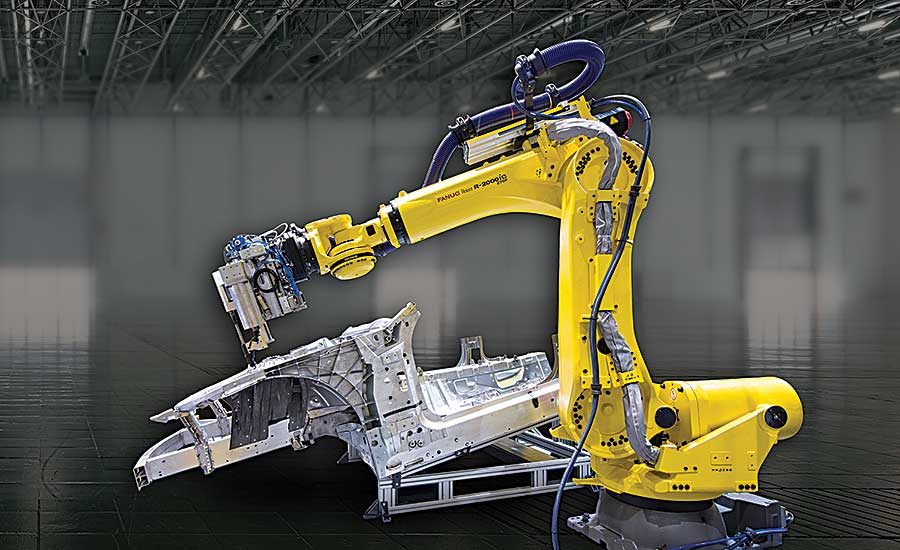This highly detailed color illustration showcases a bright yellow robotic arm, prominently positioned in the foreground of an industrial warehouse setting. The robotic arm, equipped with blue and silver hydraulics and tubing, extends several feet from its mounted base on the factory floor. It features an articulating elbow joint bent at approximately a 75-degree angle and appears to be engaged with a tool or object in its robotic hand, possibly for transporting or working on other machinery. Just behind and to the left of the robotic arm is another industrial machine, notably silver, short, and squat, sitting on a hydraulic lift-tilt ramp. The background of the illustration is blurred, giving an impression of a spacious warehouse or factory filled with open spaces and large doors, with a ceiling structure reminiscent of those found in large stadiums, enhancing the sense of scale.